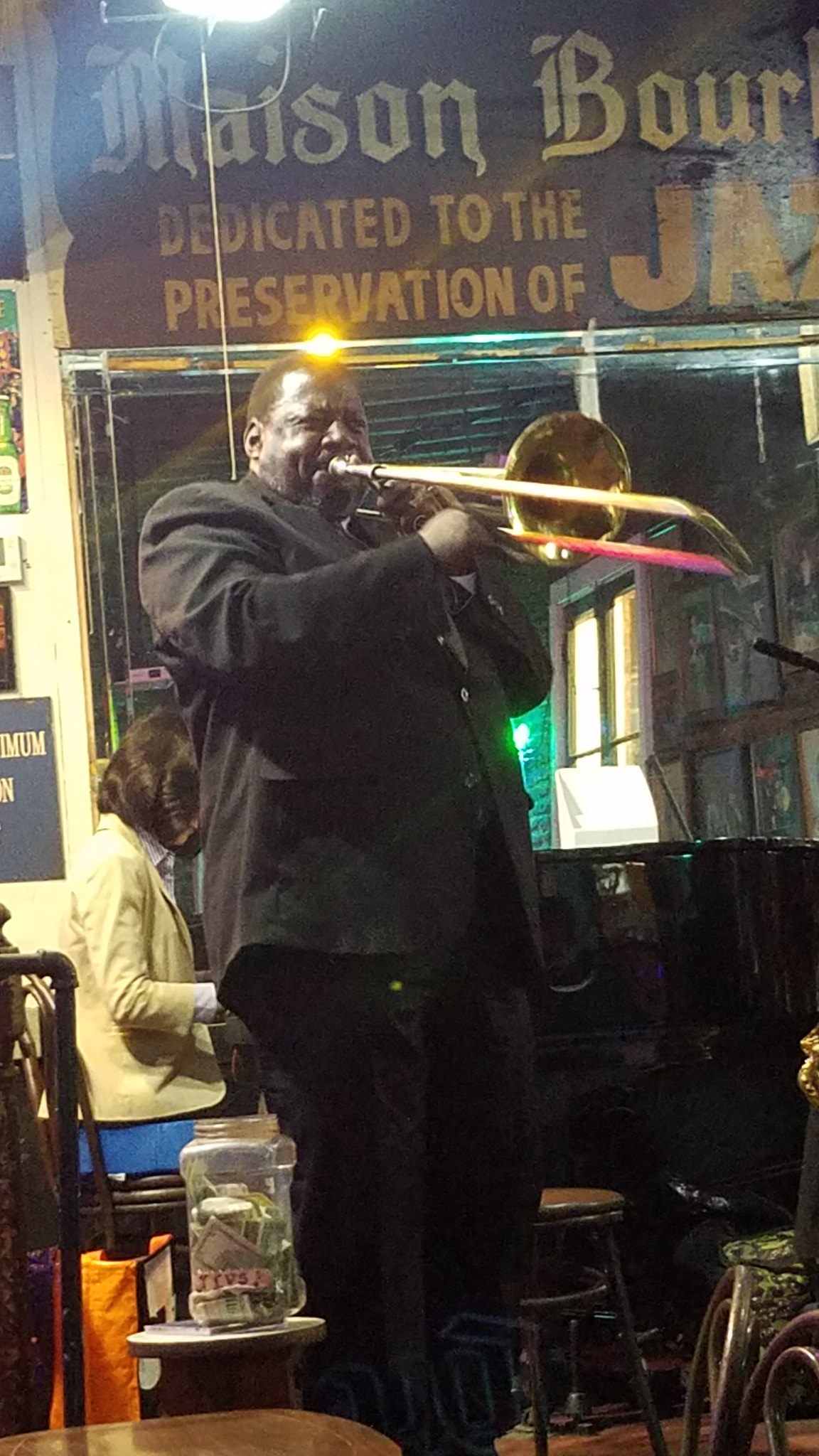In a lively jazz club cafe, a powerful African-American gentleman in a sleek black suit, engrossed in his trombone performance, takes center stage. His hands skillfully maneuver the instrument's slide. Nearby, a woman with black hair, dressed in a yellow blazer over a blue skirt or pants, attentively plays a grand piano. In front of the trombone player, a transparent tip jar brimming with dollar bills sits on a white stool with a black side. The intimate setting is adorned with various stools and small tables. A large window and a banner above it, reading "Maison Bourbon" dedicated to the preservation of jazz, set a rich backdrop. Additional details include a black chair to the left, a brown stool to the right, and a table, brown, in the bottom left corner. On the right side, there are yellow and blue bags, several signs on the wall, including a blue one with white letters partially obscured, and a mirror reflecting a door with a white frame. This image beautifully captures the essence and vibrant atmosphere of a classic jazz performance.